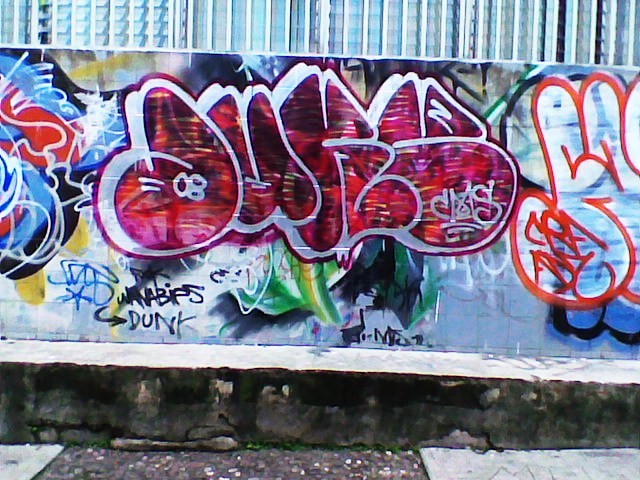This image features a graffiti-covered wall with multiple layers and textures. The top section of the wall has vertical stripes in blue, white, and black, forming a variegated pattern. Below this striped area, the bulk of the wall is dominated by heavy graffiti, with vibrant, interwoven designs that include unrecognizable and abstract letters in colors like magenta, pink, and deeper purple hues. The graffiti includes phrases like "wannabes dunk" and words like "DU" and "BIPS," though many of the inscriptions are not easily readable. A notable feature on the right-hand side is an image resembling three fingers, drawn in red with a white interior. The base of the wall consists of a white band transitioning into a stone-like step, about 12 inches high with a grayish hue along the sides. In front of this step is a sidewalk made up of mixed stone slabs, flanked by white slabs on either side. This complex artwork, rich in color and detail, epitomizes urban street art.